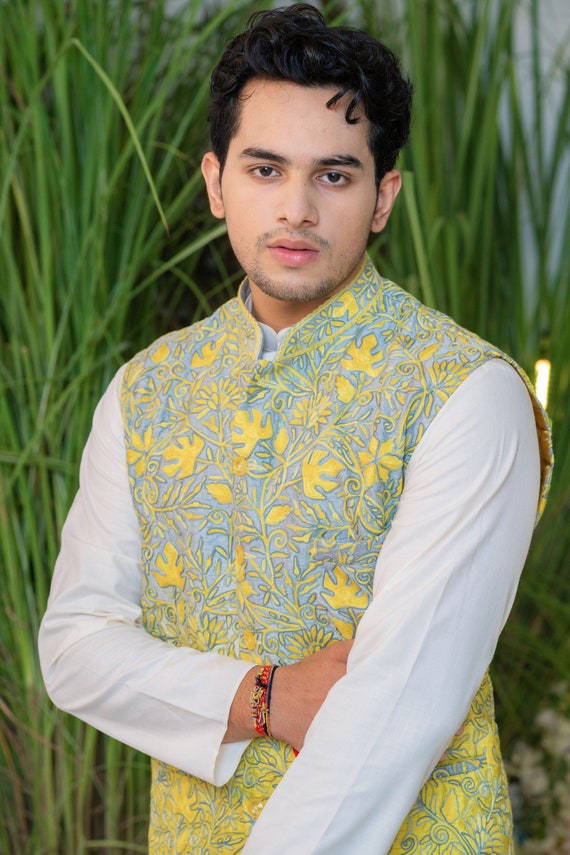The photograph depicts a young man in his early 20s, possibly of Middle Eastern or Indian descent, with slightly darker skin and dark hair styled into two small ringlets on the left side of his forehead. He has dark brown eyes and a neatly trimmed goatee, giving his facial hair a subtle, almost ephemeral appearance. His hair is about two inches long and slightly wavy, tapering towards the bottom.

The man is dressed in a striking, traditional floral vest featuring a grey background with a yellow leaf pattern, layered over a white long-sleeved shirt. He is adorned with threaded bracelets on his right wrist. His pose has his right hand positioned across his waist, while his left hand rests downward over his right.

He stands against a backdrop of tall, green reeds, appearing to be outdoors. His expression is blank as he looks directly into the camera, creating a contemplative and serene atmosphere in the image.